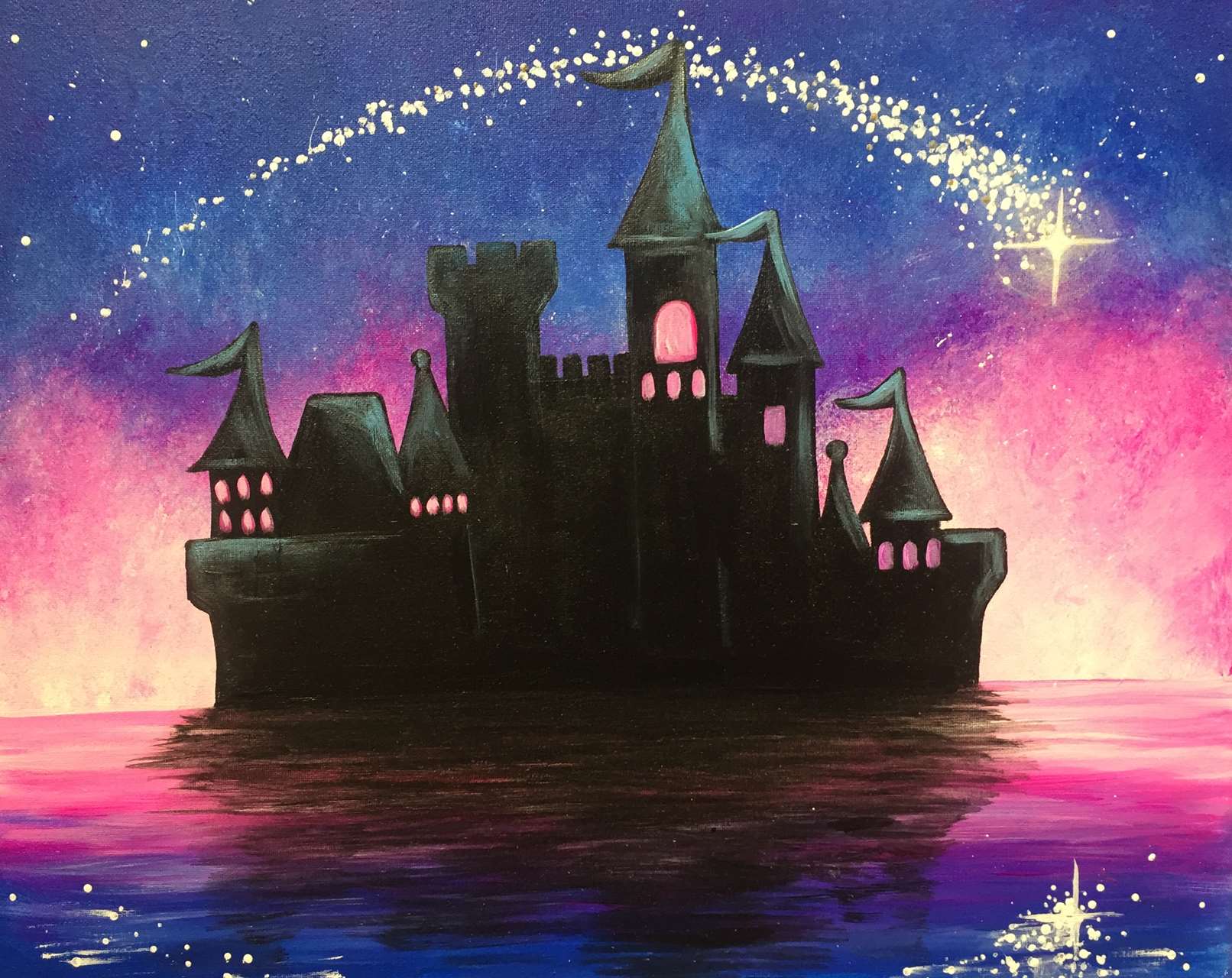In this enchanting digital artwork reminiscent of classic Disney imagery, a black castle with dark greenish-gray hues and approximately six to seven steeples stands majestically at the center. Pink light emanates from the windows, creating a magical atmosphere. Four flags proudly hang from the tips of the triangular roofs. The scene is set against a sky that transitions from deep blue at the top to a pinkish-yellow horizon, suggesting a serene sunrise or sunset. 

A twinkling white star arcs gracefully from the left to the right, leaving a trail of stardust behind it. This celestial display is beautifully mirrored in the blue water below, which also contains red highlights and star-like reflections. The water captures a dark shadow of the castle, enhancing the overall fantastical quality of the image. The vivid blend of colors, including the bright pink backdrop behind the castle, deep blues, and sparkling whites, completes this stunning and iconic visual tribute to the world of Disney.